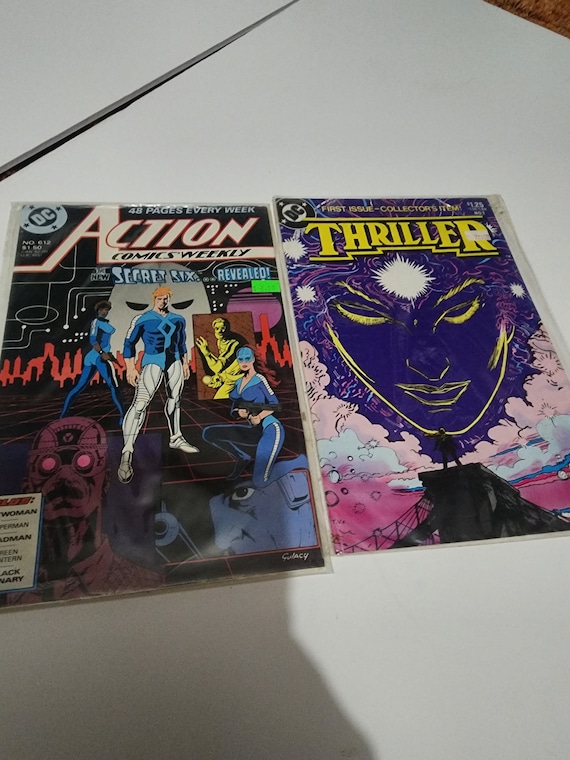This photograph depicts two vintage DC comic book covers placed side by side on a white table. The comic on the left is titled "Action Comics Weekly" and prominently features an array of superheroes. In the foreground, a female superhero clad in a blue bodysuit stands next to a male hero wearing a blue top and white tights. A yellow figure, likely a villain, looms in the background. Additional characters include a golden man at the top, a woman with blue and white attire, and a maroon man with pink eyes at the bottom left. Flames create a dramatic backdrop, giving the cover a dynamic feel. The DC Comics logo and the text "48 Pages Every Week" are visible at the top.

The right comic book is titled "Thriller," with its name displayed in bold yellow letters. This cover features a striking, blue-tinted face of a woman with yellow outlines and pink hair, a radiant white light emanating from her forehead. Below her, a man dressed in black stands atop a black tower with suspension cables, appearing to overlook a pink sea with white waves. The tagline "First Issue Collector's Item" is written above the title. Surrounding the blue face are pink clouds and a bridge, adding a surreal element to the composition. Both comics are encased in protective plastic wrappings, indicating their collectible status. Shadows from the person taking the photograph and an overhead lamp add a layer of depth to the scene.